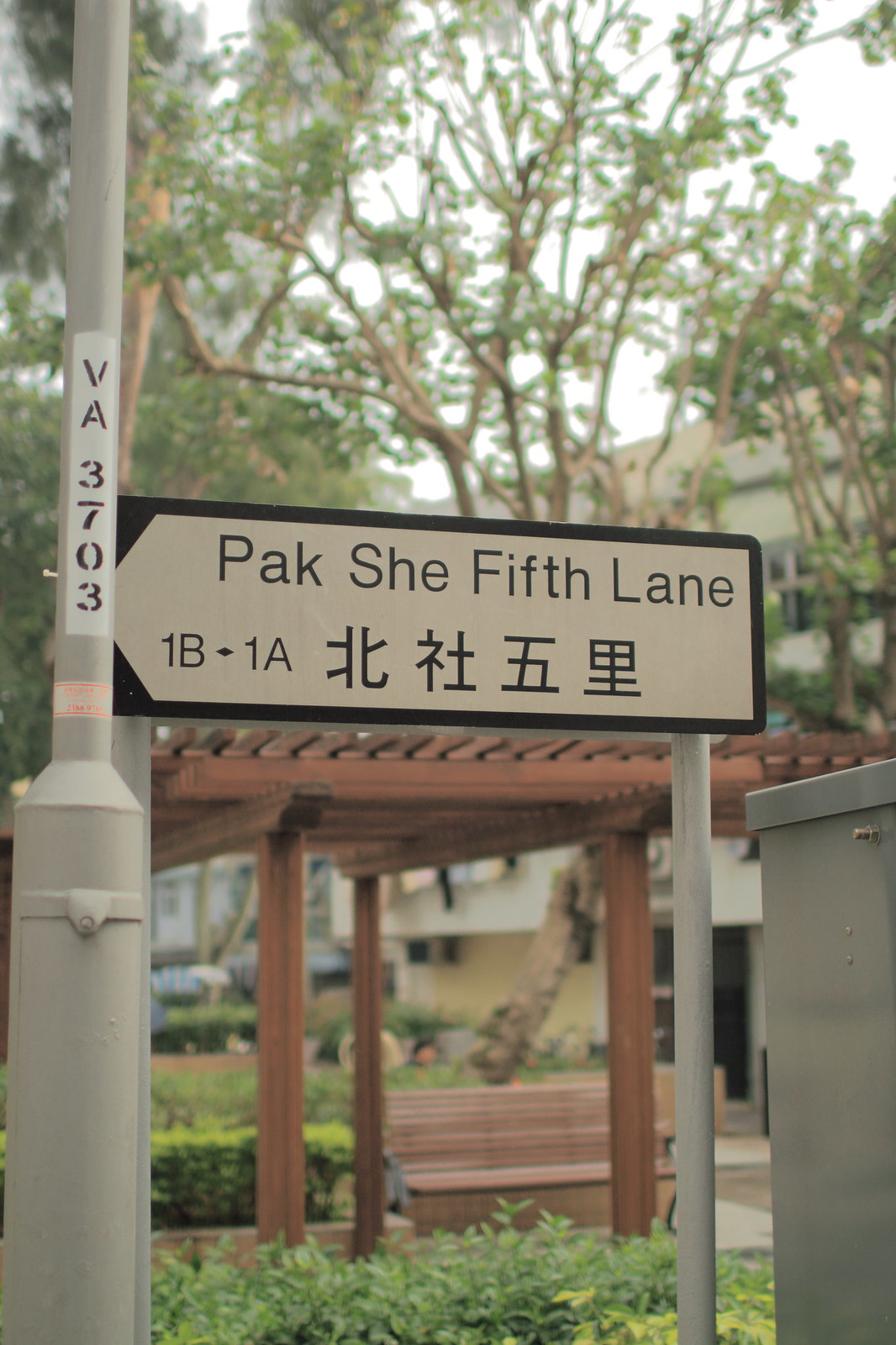In a vertically aligned rectangular photograph taken outside a street sign in a non-U.S. location, featuring symbols indicative of a foreign language, the scene unfolds with several discernible details. The upper portion of the image showcases vibrant green tree leaves with glimpses of a bright, mostly white sky peeking through the branches. In the background, a taller building with a white to tannish hue is faintly visible, along with cars parked nearby.

Dominating the left foreground, there is a light gray pole bearing a vertical inscription that reads "VA 3703" against a white background. Attached below this pole is a horizontally aligned rectangular sign bordered in dark brown with a tan background. The sign displays the text "PAC, P-A-K, she, 5th Lane" in brown letters, followed by "1B" and "1A" along with a series of four Asian symbols, likely either Japanese kanji or Chinese characters.

Adjacent to this, a black sign with white text and a left-pointing arrow is mounted on the pole, reiterating "Pac-Chi 5th Lane" along with "1B1A" and additional Asian characters. Just to the right of the sign, a small silver electrical box is visible. The setting includes a brown wooden gazebo situated on a wood frame, complemented by a brown park bench and surrounded by lush bushes. In the background, people can be seen sitting in the gazebo area, which adds a lively touch to what appears to be a park or garden-like environment.